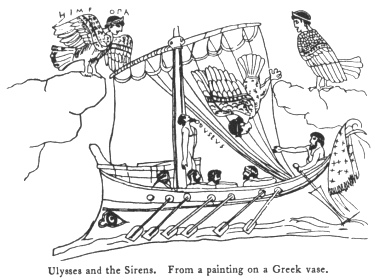This intriguing black-and-white sketch depicts a scene titled "Ulysses and the Sirens" from a painting on a Greek vase. The image shows a long ship navigating the sea, manned by four seated rowers and commanded by a figure at the ship's helm. The ship is detailed with a large sail and multiple oars on its side. Above and around the vessel, three siren-like creatures hover, each with the body of a bird and the head of a human. The leftmost creature stands on a rocky cliff with its wings outstretched, while the rightmost siren also perches on a rock, its wings tucked by its side. The central creature hangs upside down in the ship's mouth, its wings dramatically extended. Elements such as bird-like feet, tail feathers, and a bird-like design on the ship's prow add to the scene's fantastical quality. All these details combine to illustrate the mythological encounter vividly.